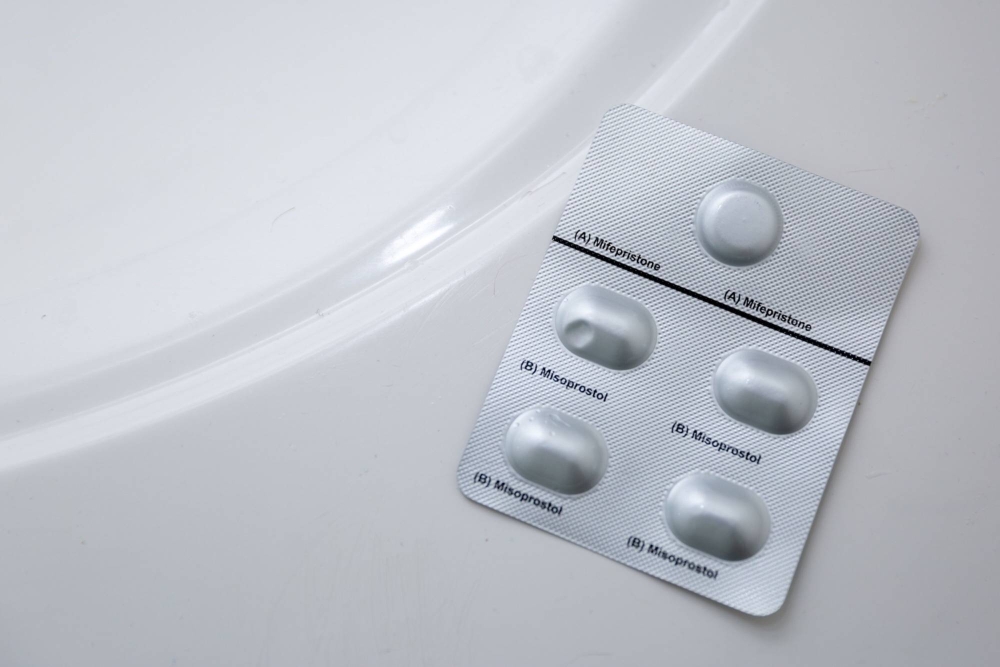The image showcases a horizontally aligned rectangular blister pack of pills placed at a diagonal angle against a light gray, possibly microwave plate background. The blister pack, predominantly silver with a fine-textured backing, contains five pill slots: one round pill at the top, and four oval-shaped pills arranged in two rows of two. The top round pill is labeled with an "A" in parentheses, followed by "Mifepristone". Below a thick black line that horizontally separates the pills, the four oval pills are labeled with "B" in parentheses, followed by "Misoprostol". The blisters themselves are silver, and the letters and names indicate different types of medication within the blister pack.